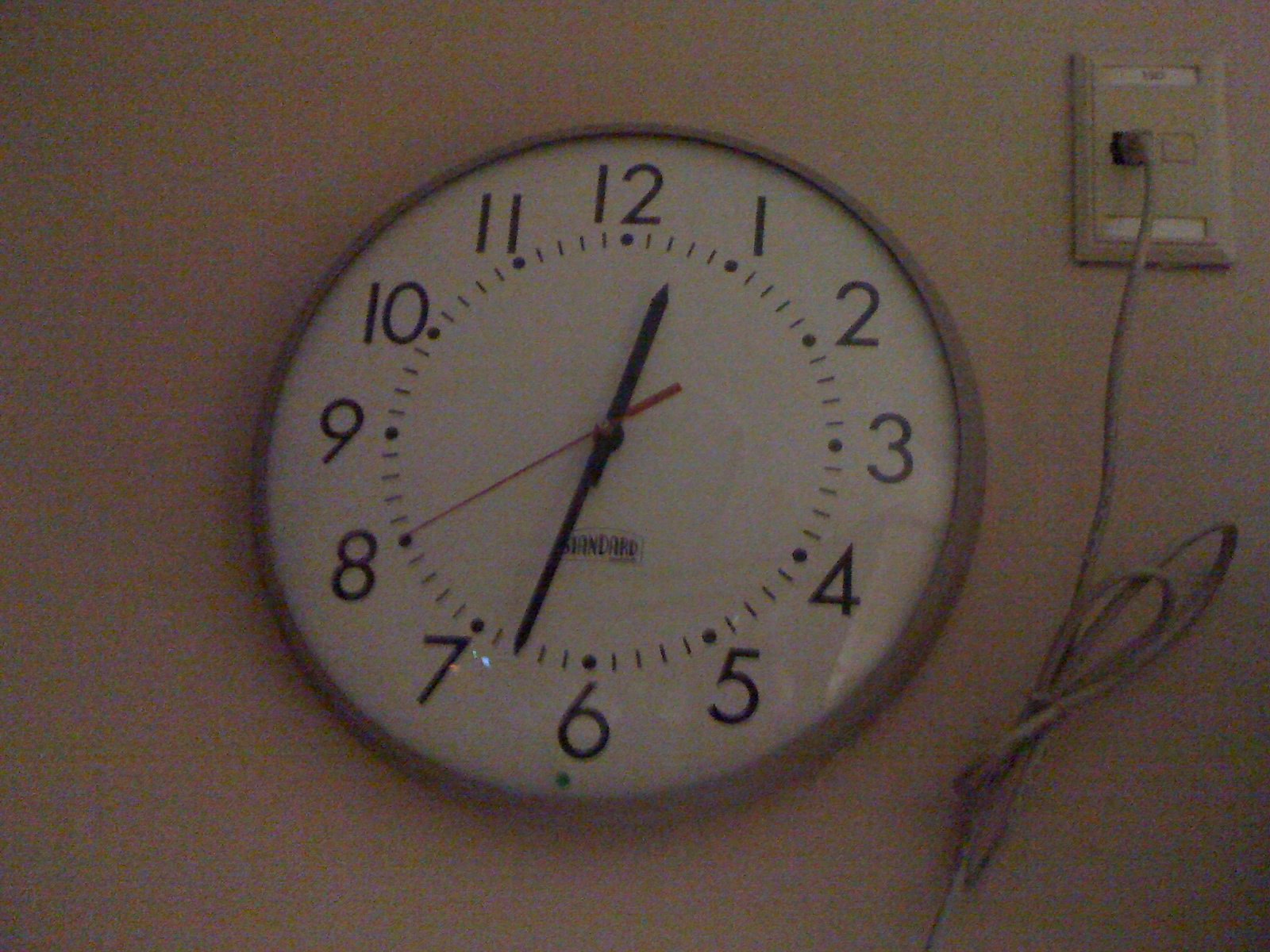This photograph features a circular analog wall clock with a gray frame, reminiscent of vintage school clocks. Despite the low resolution and granular quality of the image, the details of the clock are discernible. The clock displays bold black hour and minute hands, complemented by a vivid red second hand. Surrounding the clock face, numbers from 1 to 12 indicate the hours, each marked by a black dot above them. Slim black lines between these hour markers delineate the minutes. Below the center of the clock, a logo or label reads "Standard." Notably, beneath the number 6, there is a distinct green dot. The clock is mounted on a wall painted in a beige hue, though the exact shade is difficult to ascertain due to the image quality. Adjacent to the clock is a plastic wall plate with an electronic cord plugged into it, which does not appear to be related to the clock itself.